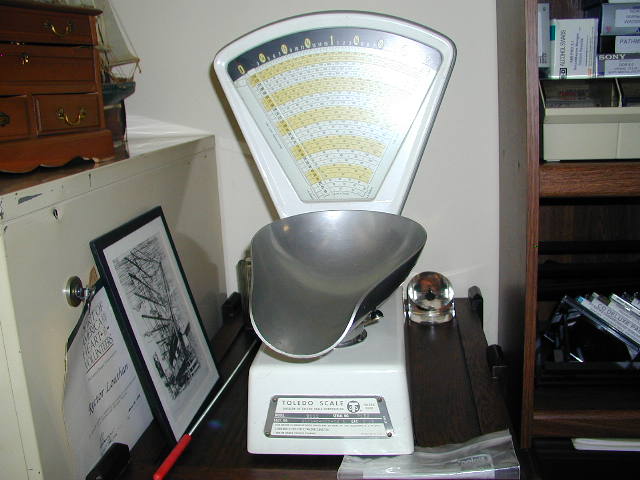In the center of the image, there is a Toledo scale reminiscent of those used in a doctor's office for weighing babies. To the left of the scale, a poster with a black border is displayed against a white background. Below the poster, a white shelf or cube is visible. At the top left corner, a small wooden mini drawer adds a touch of warmth to the scene. 

On the right side, a bookshelf houses tapes and CDs on its shelves. Nearby, a wooden table supports a metal object adorned with a red handle. Various plastic bags are scattered at the bottom of the shelf. 

The back wall is entirely white, creating a clean backdrop for these items. Additionally, a magnetic clip on the left side is holding up a piece of paper, and a small poster is seen leaning against a cabinet, completing the detailed tableau.